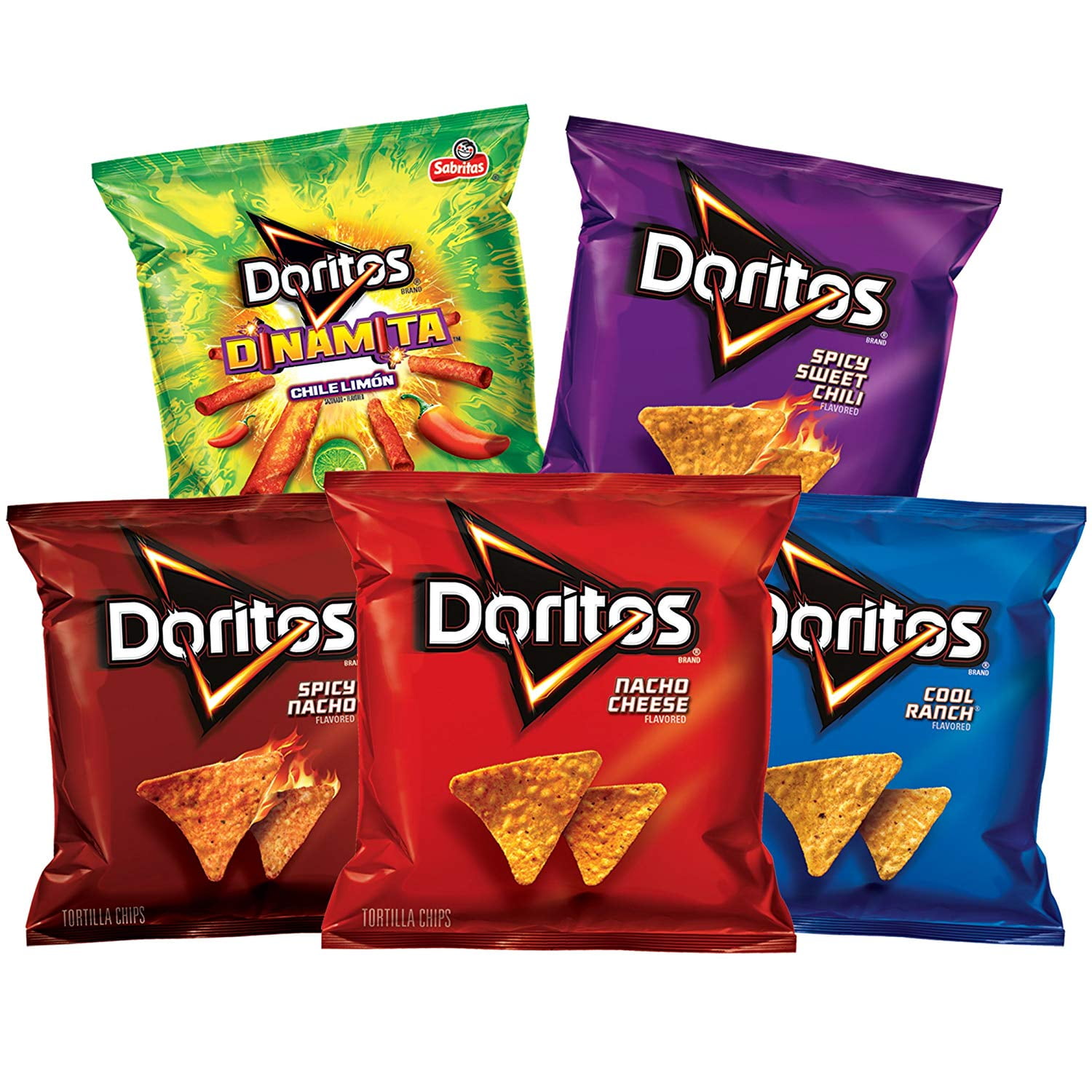This landscape-oriented color photograph showcases five assorted Doritos packaging varieties against a white, borderless background, giving the impression that they are floating. The arrangement features two bags on the top row and three on the bottom row. Starting from the top left, there is a bright green bag labeled "Doritos Dinamita," which appears to contain a candy-like product rather than chips. Adjacent to it on the right is a purple bag labeled "Spicy Sweet Chili." On the bottom left is a dark red bag marked "Spicy Nacho," characterized by the classic Doritos logo and an image of two triangular chips. Centrally positioned on the bottom row is a cherry-red bag of "Nacho Cheese," also featuring the Doritos logo and chip images, and partially overlapping the adjacent packages. Completing the bottom row on the right is a blue "Cool Ranch" bag, similarly showcasing two chips. The entire composition employs photographic realism to highlight each bag’s unique design and flavor distinction.